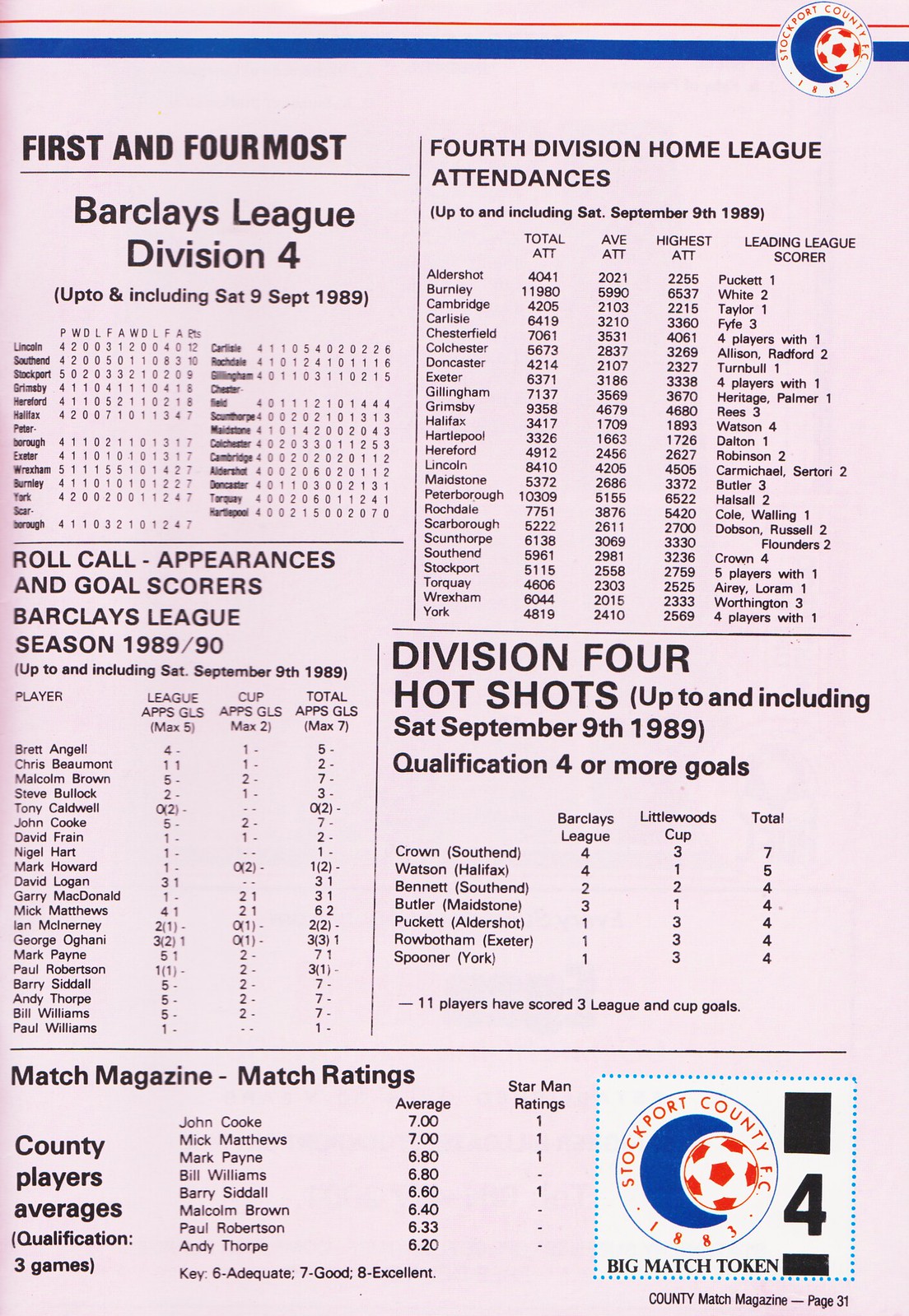This is a detailed page extracted from "Country Match Magazine," specifically from page 31, and prominently features information and statistics about Stockport County FC, highlighting their 1883-established logo, which includes a soccer ball adjacent to a blue letter "C." The same distinctive logo is positioned in both the top right and bottom right corners of the page. The top left section of the page is headlined by "Barclay League, Division 4," detailing the league statistics up to and including Saturday, 9th September 1989. Adjacent to this, the right-hand column documents the 4th Division Home League Attendances for the same date. Directly below this, the "Division 4 Hot Shots" section lists top-scoring players who have qualified with four or more goals, including names like Crown, Watson, Bennett, Butler, Puckett, Rowbottom, and Spooner. On the left side, a section titled "Roll Call: Appearances and Goal Scores, Barclay League, Season 1989–1990" offers more player statistics. The bottom segment of the page reads "Match Magazine," providing match ratings and average scores for County players, with a three-game qualification criterion. Overall, the page is rich with historical data and player performance metrics, catering to avid followers of Stockport County FC.